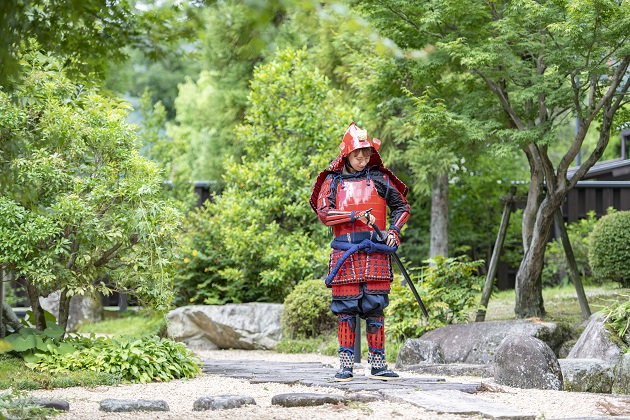The image depicts a young individual, possibly a boy, dressed in a traditional Japanese samurai costume, featuring a combination of red, blue, and white colors. He is adorned with a shiny, red helmet with flaps extending below his face, which partially obscures his features, making it hard to determine his exact identity. The costume includes a red cape and a vest-like garment, secured with a blue belt tied around his waist. The samurai attire extends into protective arm pieces and shin guards, all intricately tied with blue rope. His leggings are puffy and blue around the knees, and he wears red and white socks paired with soft-soled shoes traditional to samurai. Attached to his waist is a samurai sword that he is drawing. 

The backdrop of this photograph, which seems to be taken outdoors during the daytime, includes a variety of lush green trees with gray and brown stumps. He is standing on a rocky, stone-paved area surrounded by stones and gravel. To the far right, there is a partial view of a house. The scene reflects a natural, garden-like setting, without any additional objects or text in the photograph. The image appears to be a casual snapshot rather than a professionally taken picture.